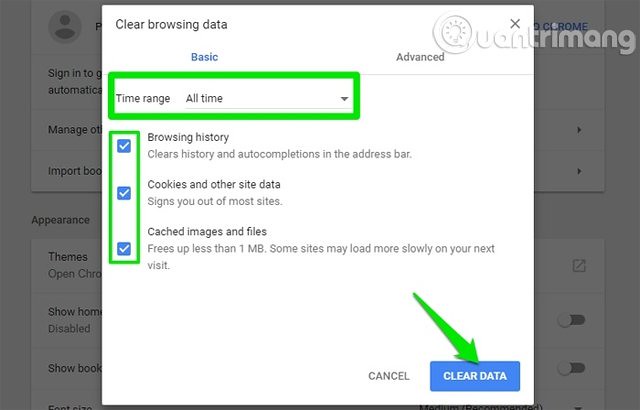The image depicts a screenshot of the Google Chrome browser's "Clear Browsing Data" settings. 

In the top left corner, there is blue text displaying "Chrome," and below it on the left, text options saying "Manage," "Import," "Appearance," "Themes," "Open Chrome," "Show," "Disable," and "Show Boops." The top right corner features text that reads "Huang Chiming, Q."

The main focus of the image is a large white dialog box situated in the top left section, labeled "Clear Browsing Data." This dialog box is divided into two tabs: "Basic" on the left and "Advanced" on the right. Adjacent is a green rectangle and further to the right is a dropdown menu labeled "Time range," currently set to "All time."

Inside the dialog box, there are three options with blue checkmarks in green rectangles next to them: "Browsing history," "Cookies and other site data" (with the note "Light gray, science most sites"), and "Cached images and files" with a description that reads, "Frees up less than one megabyte. Some sites may load more slowly on your next visit."

At the bottom of the dialog box, there are two buttons: "Cancel" on the left and a large, dark blue "Clear data" button on the right. A green arrow is pointing towards the "Clear data" button, drawing attention to it. The background of the image is somewhat blurred but indicates the Google Chrome settings interface.

Overall, the screenshot highlights the options available for clearing browsing data in Google Chrome, with a particular emphasis on the "Clear data" button.